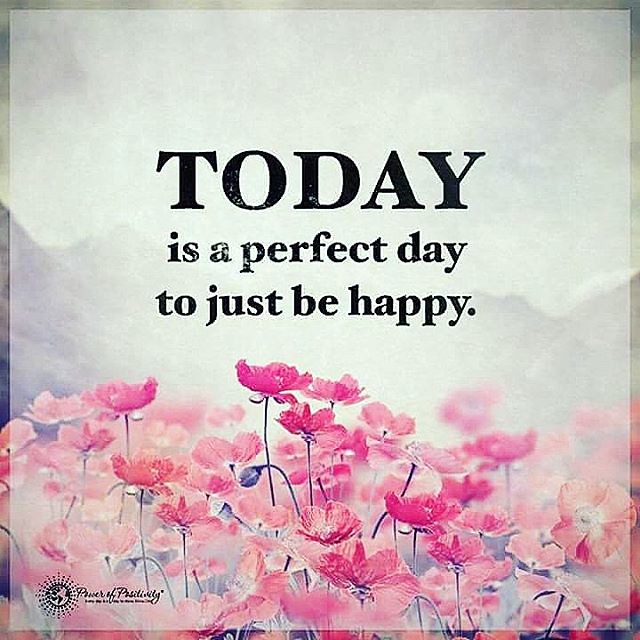The image appears to be an old, possibly decades-old, scanned or screenshot poster that now shows significant JPEG artifacts, suggesting it might have been originally from a magazine or similar publication. The central message, written in black text, reads: "Today is a perfect day to just be happy," with "today" in all capital letters. This positive message is superimposed over a mostly blank sky backdrop that has a hint of mountains in the far distance.

The bottom half of the image features a close-up of a field of small, reddish-pink and white flowers, some of which haven't bloomed yet, giving a lively and serene visual emphasis. In the lower left-hand corner, there is a "Power of Positivity" logo, which includes a drawing of the Earth with radiating lines, suggesting a focus on spreading positive vibes. Overall, the picturesque scene, combined with the heartening message, successfully delivers a mood-lifting and aesthetically pleasing visual experience perfect for social media sharing.